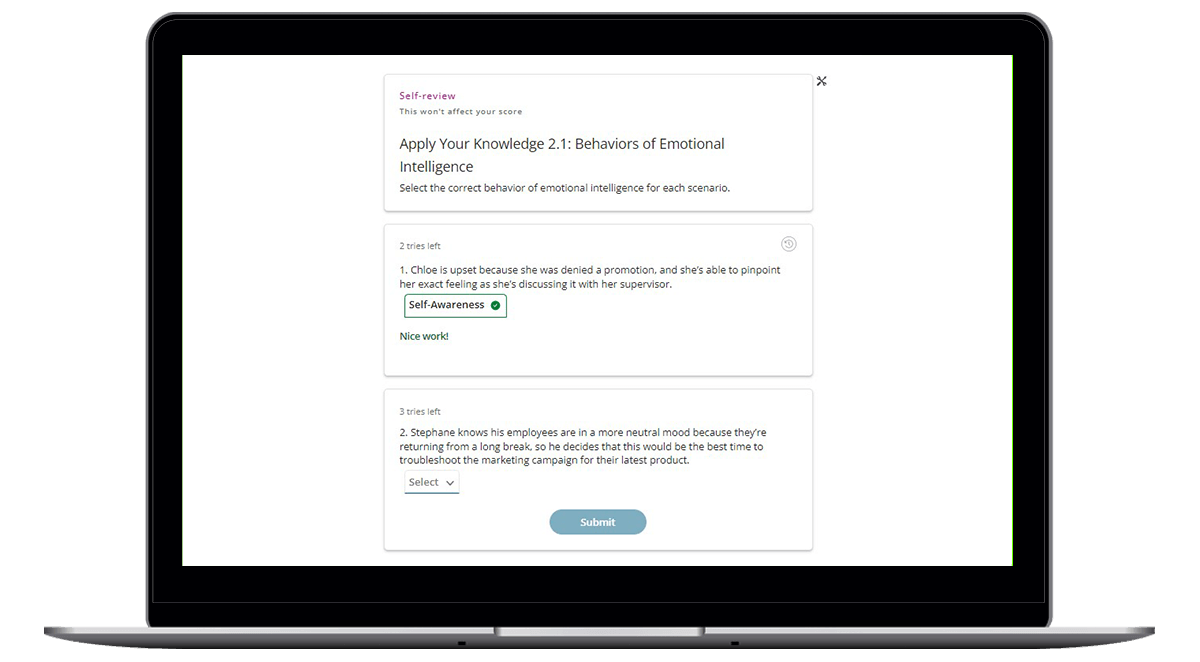The image captures the screen of a silver laptop, viewed from an angle that allows you to see the external frame and the display. The base of the laptop is silver, while the bezel surrounding the screen is black and approximately an inch thick, indicating it's not one of the ultra-thin designs. The screen displays a webpage with a predominantly white background. 

At the top-right corner of the webpage, there's an "X" button for closing the window. Below that, the webpage is titled "Self-Review. This won't affect your score." The content focuses on identifying behaviors of emotional intelligence, with interactive elements that invite users to select correct behaviors for each scenario. 

One scenario describes Chloe, who is adeptly aware of her emotions after being denied a promotion and discusses her feelings with her supervisor, demonstrating "Self-awareness." Another scenario involves Stefan, who recognizes his employees are in a neutral mood after returning from a long break and decides it's an optimal time for troubleshooting a marketing campaign, with the answer to be selected via a dropdown menu. The interface includes a blue "Submit" button for submitting responses.